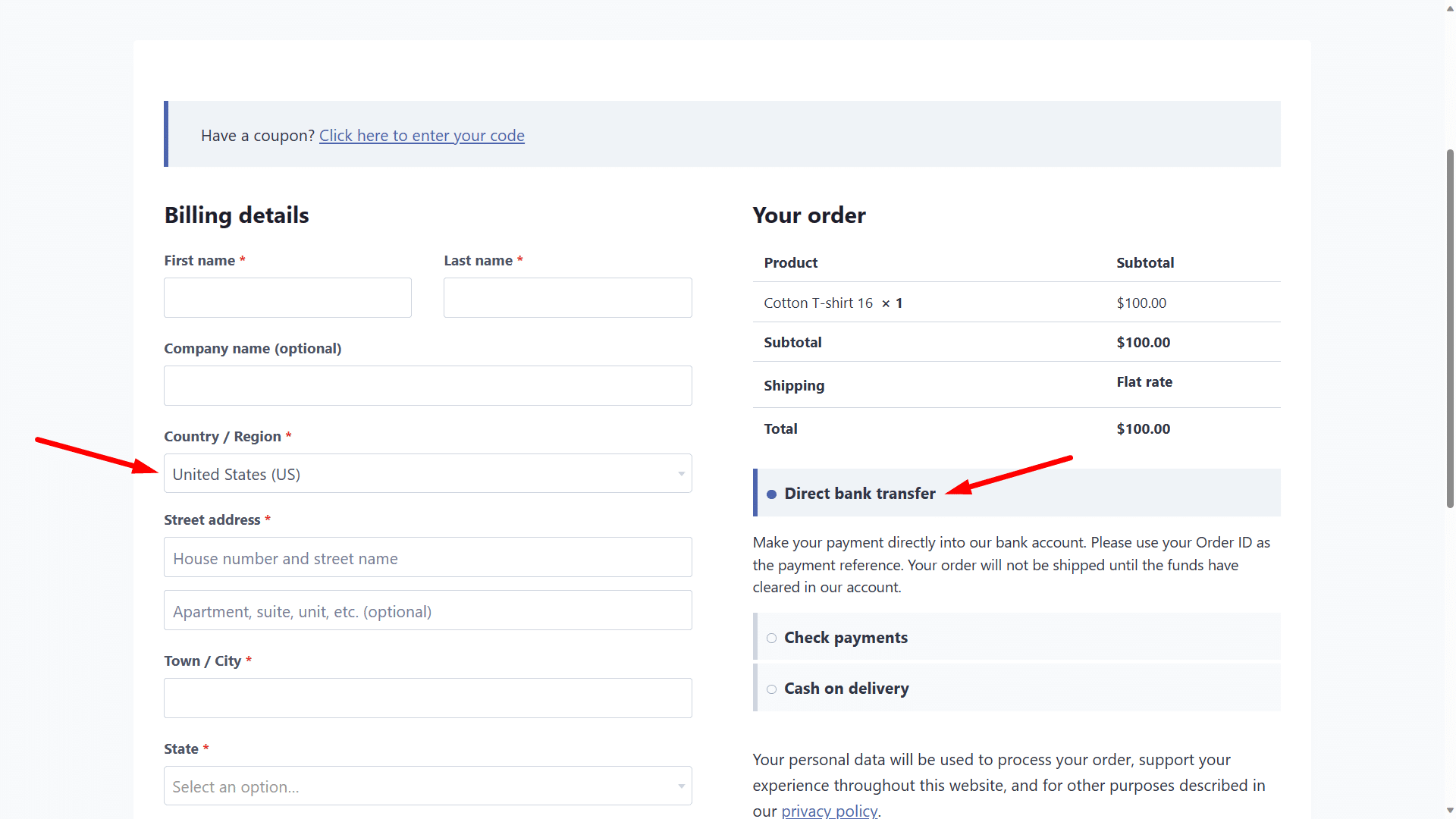The image displays an online checkout page with a structured layout. The background transitions through three sections: a light gray top section, a middle white section, and a bottom light gray section again. 

On the left, a blue line highlights a feature where "Have a coupon?" is written in black font, followed by a clickable underlined blue text, "Click here to enter your code."

Below this, in the white section, the heading "Billing details" is displayed in black font. The billing information form fields follow, each accompanied by a red star indicating a required field:
- First Name: with a gray input box
- Last Name: with a gray input box
- Company Name (optional): in gray text, with a gray input box
- Country/Region: defaulting to "United States" in a selectable gray box, highlighted by a red arrow

Further fields include:
- Street Address: with placeholder text "House number and street name" in a gray box, and "Apartment, suite, unit, etc. (optional)" in a subsequent gray box
- Town/City: with a gray input box
- State: with a drop-down selection gray box, indicating "Select an option" and trailed by a downward arrow

On the right, the "Your order" section itemizes the purchase:
- "Product" and "Subtotal" headings separated by a gray line
- "Cotton T-shirt (x15): $100"
- Subtotal: "$100"

Below this, the shipping method is labeled "Shipping - Flat rate," followed by the total cost of $100.

Payment options are detailed:
- "Direct Bank Transfer," indicated by a blue dot and blue line, with an accompanying red arrow emphasizing it. Below, instructions are in gray font, stating to "Make your payment directly into our bank account. Please use your order ID as the payment reference. Your order will not be shipped until the funds have cleared in our account."

Finally, two additional payment methods are listed, each within gray-lined boxes:
- "Check payments" with a gray circle
- "Cash on delivery"

At the bottom, in gray font, a privacy notice reads: "Your personal data will be used to process your order, support your experience throughout this website, and for other purposes described in our privacy policy," with "privacy policy" underlined in blue for emphasis.